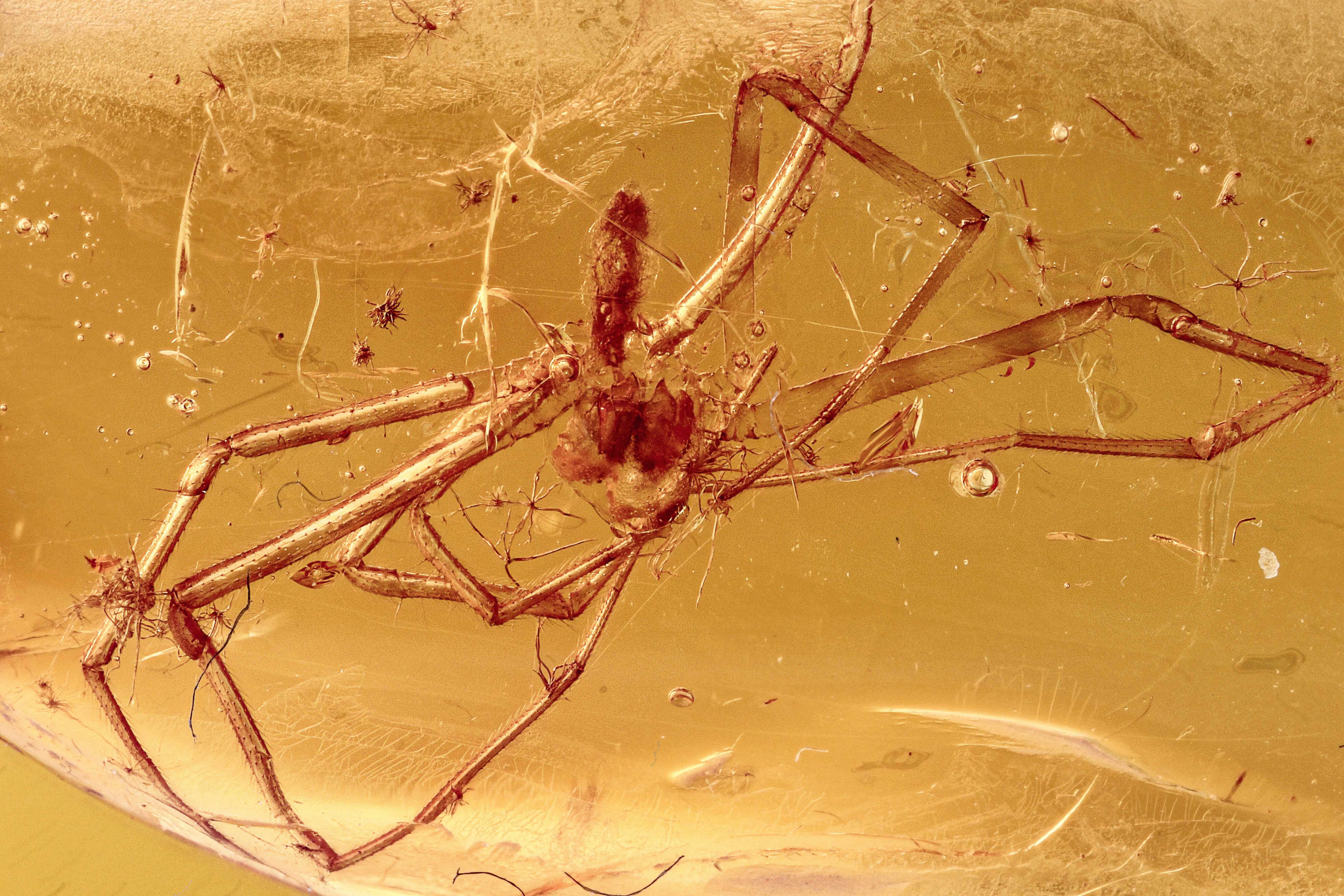The image depicts a close-up view of a large, deceased spider, possibly preserved or encased in some sort of translucent material that has helped maintain its shape over time. The background is a light brownish-beige, resembling a faded, scratched surface, with hints of what could be webbing around the spider. The spider's long legs are intricately curled inwards and its body, although somewhat eroded and indistinct, still showcases its hairy texture. The entire scene has an almost surreal, artistic quality, making the spider appear as though it's trapped within a delicate, capsule-like structure, giving a sense of a specimen from the past preserved for eternity.